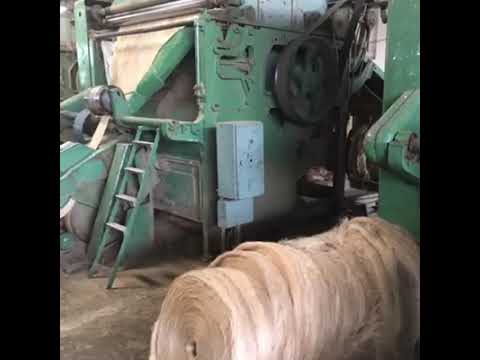This image showcases a large, rectangular green machinery unit in a factory setting. Attached to the left side of the machinery is a green ladder, leading up to an accessible area on the machine. Prominently, there is a big, spoked black wheel and other black mechanisms that appear to be part of a pulley system. On the right side of the machine, partially visible, is another piece of green machinery.

In the foreground, there is a notable feature: a large spool, several feet in diameter, of what looks like plastic wrap or a similar material, likely being processed or produced by the machinery. The spool appears light brown or white. Additionally, there is a light blue box situated to the right of the main machinery unit, contributing to the overall industrial environment. The factory floor is a dark brown, indicating a well-used workspace. The image emphasizes the machinery's potential role in spooling and wrapping materials, integral to the factory's operations.